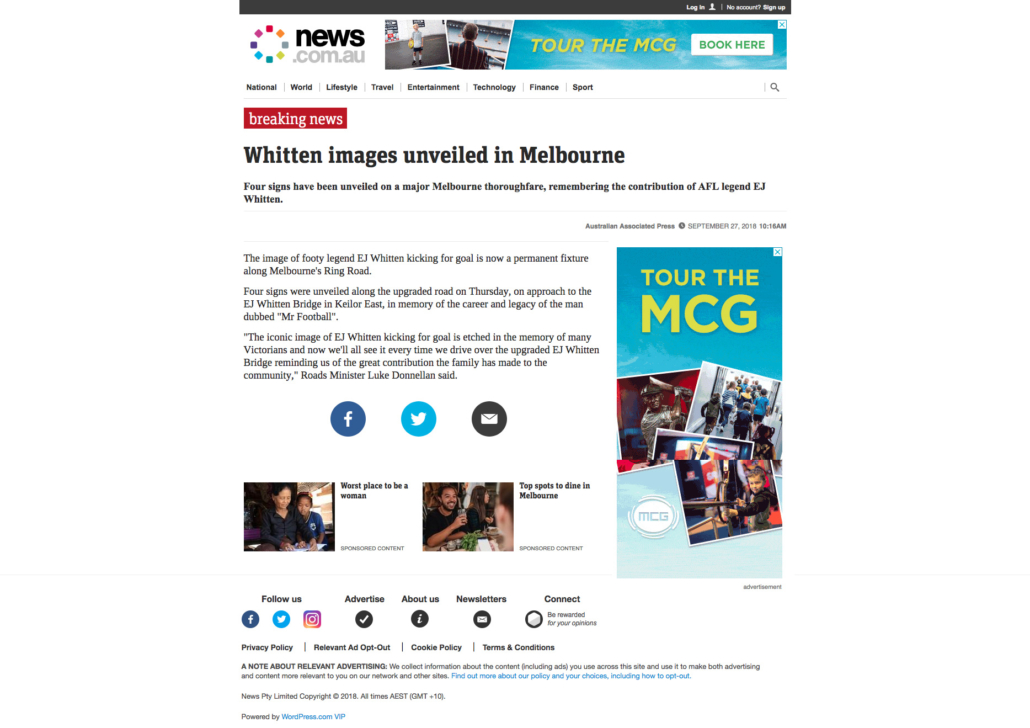**Detailed Caption:**

The image captures a screenshot of a web page from "news.com.au." At the top of the page, there is a navigation menu that includes icons and images, including one of a boy holding a basketball and another of a man seemingly watching a sports event. Prominently featured is an offer to "Tour the MCG" with a white button containing green text that reads "Book here." In the top right corner, there's an area for user login.

Positioned beneath the "news.com.au" logo on the left, a navigation bar lists various categories: National, World, Lifestyle, Travel, Entertainment, Technology, Finance, and Sport. Just below this, a red rectangle labeled "Breaking News" draws attention to the headline: "Witten Images Unveiled in Melbourne." This headline reports that four signs commemorating AFL legend EJ Witten have been installed along a major Melbourne thoroughfare.

Further details below the headline describe Witten's permanent recognition on Melbourne's ring road, highlighting that the road signs were unveiled on Thursday. On the right side of the page, there's another promotional area for touring the MCG, distinguishable by its teal background. Additionally, this section includes clickable icons for various social media platforms.